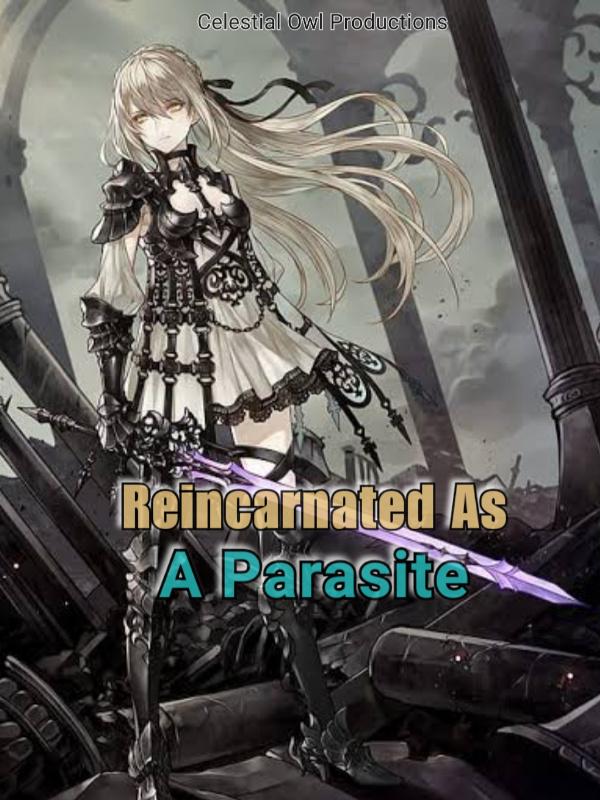Promotional Poster for an Anime Film by Celestial Owl Productions

This rectangular, vertically oriented advertisement presents a subtle yet striking visual aesthetic, leveraging a palette of almost monochromatic, pale hues that stop just short of black and white. Centered at the top in bold, black lettering reads "Celestial Owl Productions." Lower on the poster, the phrase "Reincarnated as" is displayed in a soft tan color, immediately followed by "A Parasite" in light blue letters, creating a distinctive contrast.

Dominating the left side of the poster is a tall Japanese anime girl characterized by her wavy blonde hair and vibrant red-orange eyes. She is dressed in a contrasting white and black outfit that stands in sharp relief against the backdrop. The scene behind her is an apocalyptic landscape filled with wreckage, evoking a sense of desolation and chaos.

In her hands, the anime girl wields an intricately designed, ornamental sword of impressive length, adding to the overall dramatic flair. The sky above is an unusual pale green, dotted with scattered clouds, further contributing to the eerie, otherworldly ambiance of the scene. This detailed composition effectively conveys the theme and tone of the anime, hinting at a captivating story set in a dystopian world.